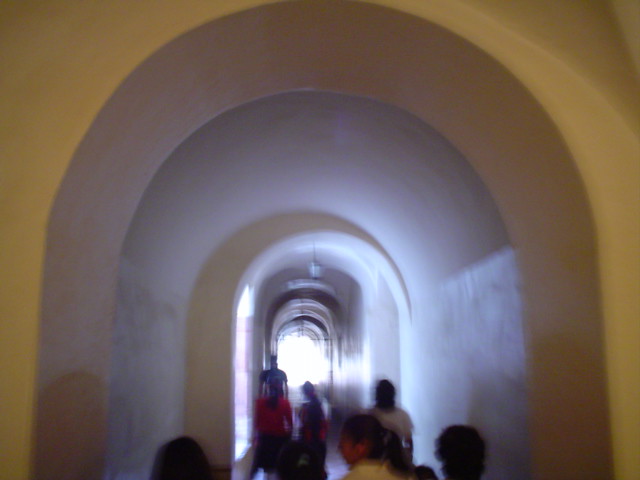The image captures a bustling, arched hallway bathed in natural light streaming through a window at its far end. The hallway, resembling a bright tunnel with shiny white walls, features pendant lights hanging from the ceiling, casting intricate shadows. The scene is slightly blurry but teems with activity; numerous people, predominantly female, are walking through. Notably, a very tall man stands out near the window at the back. Among the crowd, two females with ponytails are noticeable: one in a red shirt and another in a yellow shirt positioned in the foreground, alongside several children. The combination of artificial and natural light creates a vibrant play of reflections and shadows in the lively passageway.